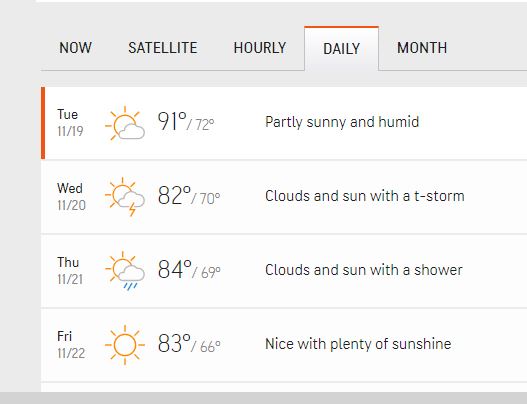This image showcases a weather report interface with a gray sidebar on the left and a gray header across the top. The header displays navigation options: "Now," "Satellite," "Hourly," "Daily," and "Month," with the "Daily" tab being highlighted in red. The report is centered around Tuesday, November 19th, indicated by a red underline.

The weather forecast for the week is displayed in white boxes as follows:

- **Tuesday, November 19th:** Partly sunny and humid with a high of 91°F and a low of 72°F.
- **Wednesday:** A mix of clouds and sun with a thunderstorm, reaching a high of 82°F and a low of 70°F.
- **Thursday:** Partly cloudy with occasional showers, temperatures peaking at 84°F and dipping to a low of 69°F.
- **Friday, November 22nd:** Plenty of sunshine, no clouds, with a high of 83°F and a low of 66°F, described as "nice with plenty of sunshine."